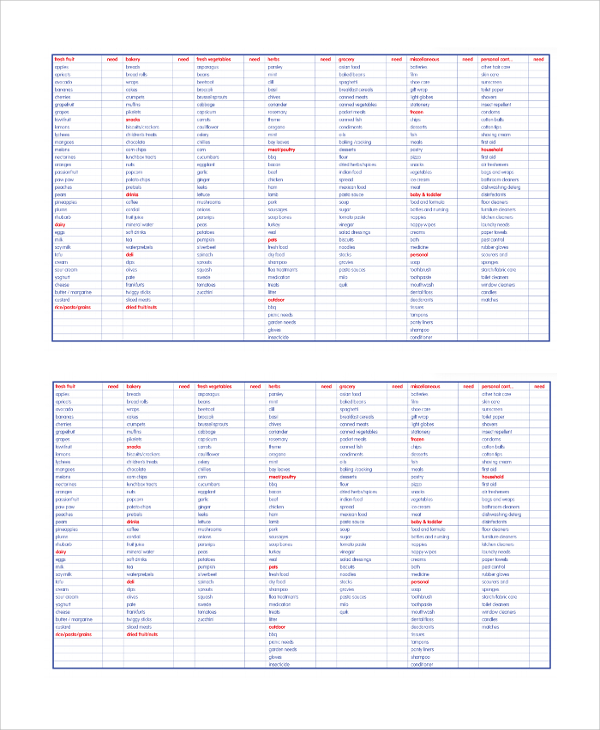The image depicts a meticulously organized, blue-tinted grid resembling an Excel spreadsheet. The grid is divided into two main vertical sections, each enclosed by a blue border, set against a plain white background. Within each main section, there are numerous smaller sub-sections. Specifically, the top section consists of 20 distinct sub-sections, each separated by red lettering, making it visually prominent. The lettering predominantly appears in blue, structured into columns that are hard to decipher due to their minute size. 

The text includes possible category labels such as "dairy" and what appears to be various grocery items, suggesting that the grid might function as a shopping list or inventory. The bottom section mirrors the top with a similar layout but contains 19 sub-sections. Overall, the intricate detailing and organized nature of the grid evoke the meticulousness of data organization or item categorization within a list-based system. The minute size, however, makes it challenging to read and interpret the precise content of the text.